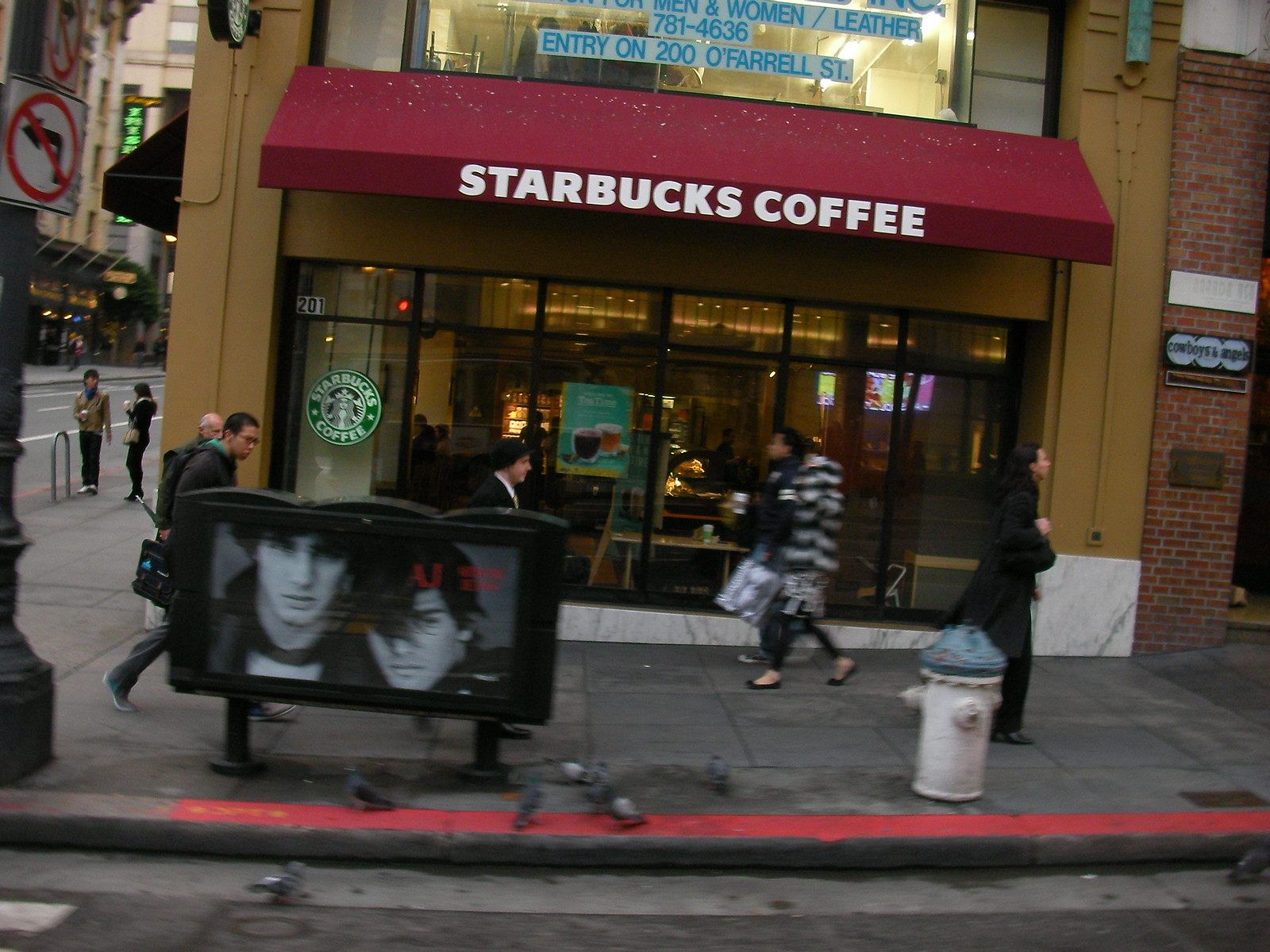The photograph captures the exterior of a Starbucks coffee shop located on a city street corner, possibly in New York. The storefront is encased entirely in large windows, adorned with the familiar Starbucks emblem. The deep maroon awning prominently displays "Starbucks Coffee" in white lettering. The image is slightly blurred and skewed, perhaps taken from a moving vehicle. Two females, dressed warmly, stroll briskly past the storefront while two males walk in the opposite direction on the gray, somewhat grimy sidewalk. The photograph also reveals a white fire hydrant with a gray top situated on the sidewalk. The inside of the Starbucks is faintly visible through the windows, showing tables, bench seats, and a screen displaying some content. In the foreground of the sidewalk, a sign with an advertisement featuring two faces is noticeable. Another shop's upper facade can be glimpsed in the background, which reads, "Men and Women Leather 7814636, entry on 200 O'Farrell Street." A red brick column, possibly part of an adjacent shop, appears on the right side of the image. Additionally, a signpost and more pedestrians and buildings are visible towards the left.